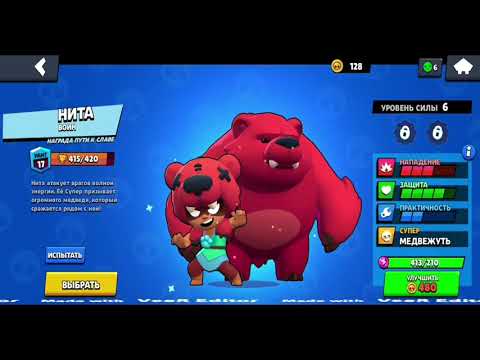This image appears to be a screenshot from a children's video game displayed on a computer screen. The screen is framed by black bars on the top and bottom, with a gray home button featuring a white left-pointing arrow located in the upper left corner. Further to the right, there is a coin icon beside the number 128 in white, and a green smiley face with the number 6 next to it. Central to the image is a large, cartoonish red bear, reminiscent of Pixar's animation style. Standing in front of the bear is a short, child-like character adorned in a bear helmet with white eyes and a green dress, appearing to be mid-pose. Additional character stats and various UI elements are scattered around the screen, including greens, blues, and reds, indicating different numeric values. The text throughout the image is written in Russian, making the specifics of the game's content challenging to decipher, but it seems to be a whimsical and colorful game interface, likely explaining various character stats and in-game points.